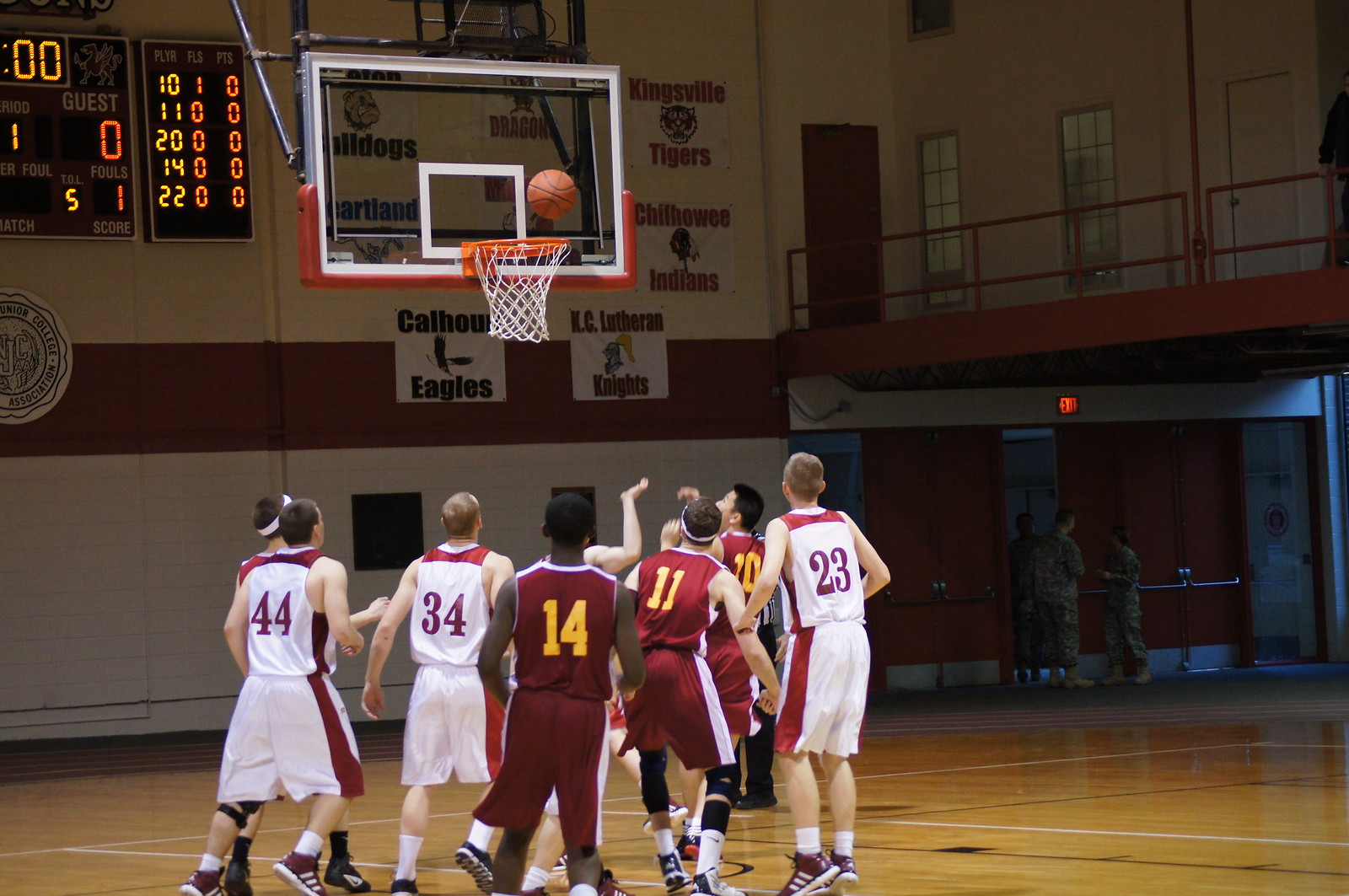This image captures an intense moment in a basketball game set in a dimly-lit gymnasium with a shiny, hardwood court marked with black and white lines. The focal point is a basketball suspended mid-air, poised just above the hoop. Surrounding the basket, players from two all-male teams are readying themselves for a rebound. One team is clad in white uniforms with red trims, while the opposing team wears maroon uniforms with yellow numbers. Behind the hoop, a scoreboard with yellow and red digital text is visible, flanked by banners of Bulldogs, Dragons, and Tigers. The gymnasium also features white walls with a red border, and in the background near the gymnasium doors, some individuals and additional banners can be seen. The poorly lit ambiance casts shadows across the scene, adding to the tension and anticipation as the ball hovers over the basket.